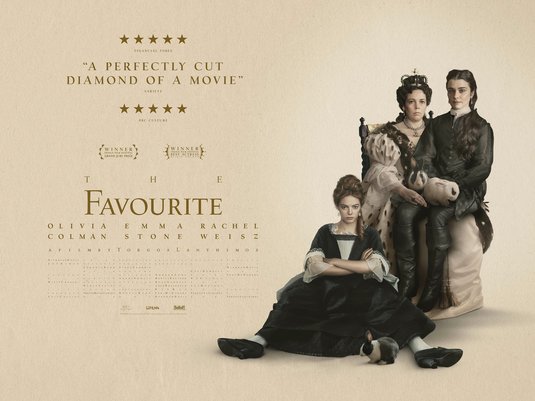The movie poster for "The Favorite," starring Olivia Colman, Emma Stone, and Rachel Weisz, features a beautifully detailed 19th-century theme against a gradient tan background. The top of the poster showcases five stars, accompanied by text that reads "A perfectly cut diamond of a movie." Highlighted accolades and awards flank the left side of the image. On the right, three key characters are dressed in elaborate black attire, evoking a historical and regal aesthetic. The central figure, likely a queen, sits on a throne wearing a crown and a dress with puffy sleeves. On her lap rests another woman, dressed entirely in black with a high collar and dark hair. At their feet, a third young woman sits on the ground with her legs spread and arms crossed, dressed in a black dress with distinctive white ruffled sleeves. A small bunny sits in front of her, adding a quaint touch to the composition. All characters exude a sense of elegance and refinement, reflective of the movie's period setting.